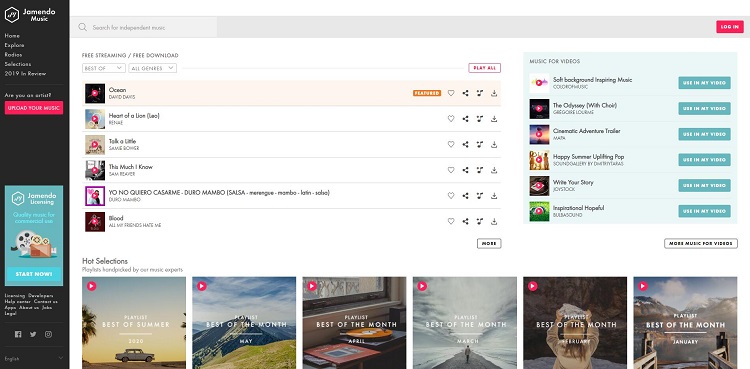The image depicts a music-centric website with several distinct sections and features. At the top, the website name appears to start with a 'J' and end with an 'O,' although the exact name is unclear. Below the title is a tagline or description that reads "This is music." To the left side, there is a hexagon-shaped logo with a 'J' in the center. Beneath this are navigation options labeled "Home" and "Explore," followed by three lines of blurred, unreadable text.

On the right side, there is a prominent red rectangular button labeled "Upload Your Music," followed by a long blue rectangular button that says "Start Now." Adjacent to these buttons are various computer-generated media icons.

Towards the bottom of the website, there are social media icons for sharing content. Below these icons is a list of songs, with the first song titled "Ocean" highlighted. There are five more songs listed underneath, each accompanied by relevant media images.

Additional options for interacting with the music, such as favoriting, sharing, and downloading, are available, displayed as heart icons, share icons, and download icons respectively.

At the bottom, there are six playlists, each with media images depicting outdoor scenes, such as mountains. Above these playlists, the text reads "Music for Videos," followed by six rows of video thumbnails, each with aqua-blue rectangular buttons beside them on the right.